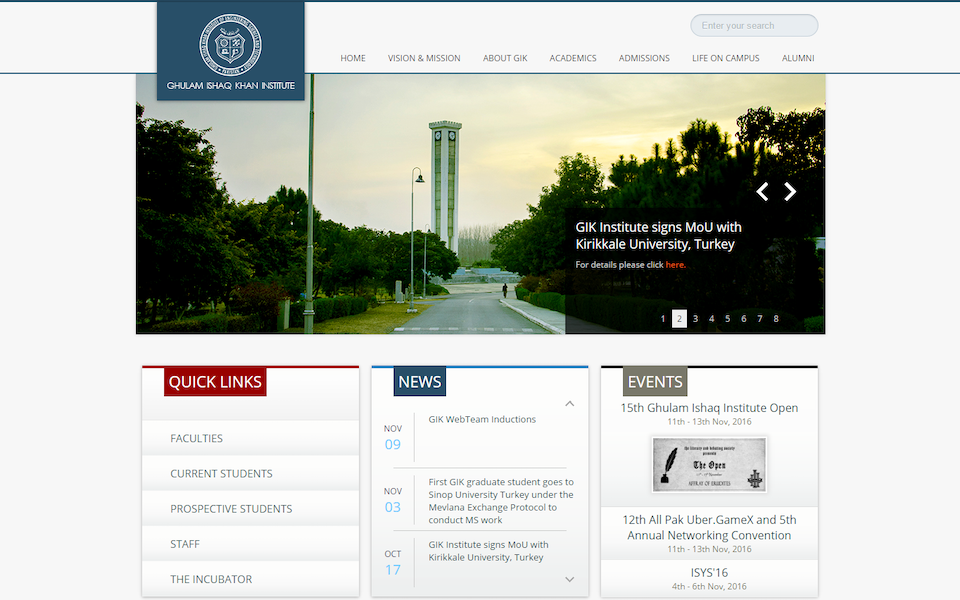**Homepage of GK Institute's Website**

This detailed homepage of the GK Institute's website features a prominently displayed logo, with text underneath written in a non-English language. At the top, the navigation bar includes the following options: Home, Vision and Mission, About GK, Academics, Admissions, Life on Campus, and Alumni.

A large central image showcases a picturesque scene with a wide road lined by sidewalks and trees on either side, leading to a tower, creating a grand entrance view. Users can navigate through this dynamic image carousel, which comprises a total of eight pages, with the current view being on page two. 

An important announcement is highlighted: "GK Institute signs MOU with Kirkcale University, Turkey. For details, please click here," with "here" hyperlinked in red. Below this, there are quick links organized into tiles covering Faculties, Current Students, Prospective Students, Staff, and the Incubator.

The website also includes a News section, featuring the following updates:
- November 9th: GK Web Team Introductions.
- November 3rd: First GK graduate student goes to SINOP University, Turkey, under the Melvia Exchange Protocol to conduct MS work.
- October 17th: GK Institute signs MOU with Kirkcale University, Turkey.

Additionally, there is an Events section listing three upcoming events, ensuring that visitors can stay informed about recent and future activities at the institute.